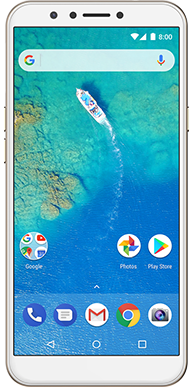The image features a white smartphone, likely a Google Pixel or Samsung device given the strong presence of Google applications, rather than an iPhone. The phone’s screen displays a vibrant home screen with a prominent Google search bar at the top. The background image is a stunning, top-down photograph of a boat cruising through crystal-clear teal blue waters, revealing the ocean floor beneath dotted with brown and tan rocks or possibly coral, reminiscent of Caribbean waters. At the bottom of the home screen, icons for phone call, text messaging, Gmail, Google Chrome, and the camera are neatly arranged. Above these, icons for the Play Store, Google Photos, and various other Google apps are displayed, emphasizing the device's Android nature.